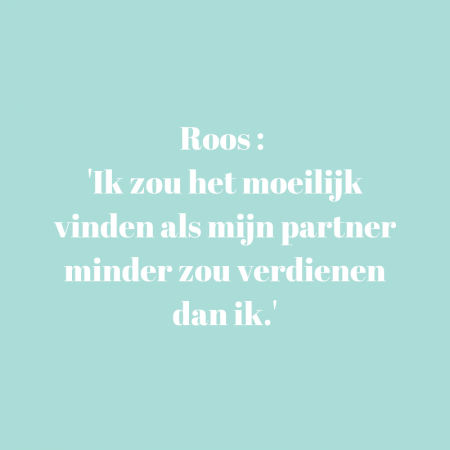The image features a solid light blue background with slightly bold, white text resembling a clean, modern font such as Century Gothic. In the center, there is a quote in a foreign language using English letters, presented in five lines. The first line starts with "Roes:" followed by the text, which reads: 

"'Ik zou het moeilijk vinden als mijn partner minder zou verdienen dan ik.'"

The text is enclosed within single quote marks at both the beginning and the end, emphasizing the quote format.